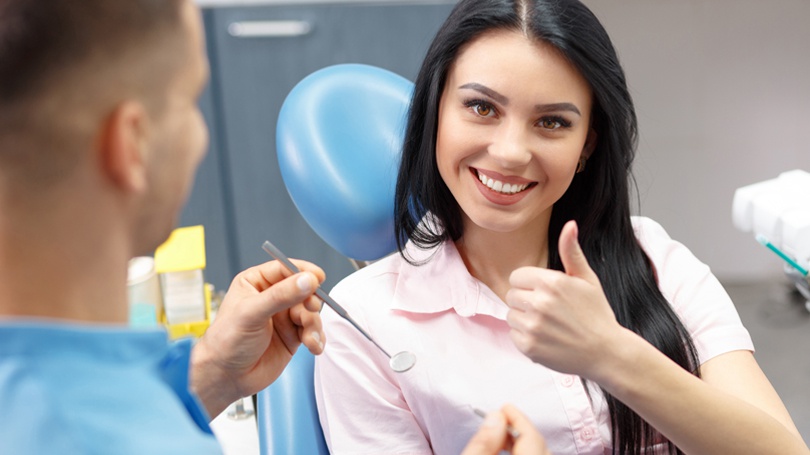This detailed photograph captures a cheerful moment in a dentist's office, featuring an attractive woman seated in a dental chair with a thumbs-up gesture. The chair, including a light blue headrest, provides a backdrop for her exuberant expression. She sports a light pink, short-sleeved collared button-down shirt and has long, straight, black hair parted in the middle. Her brown eyes and dark brown eyebrows frame a brilliant smile showing off her white teeth. To the left, partially captured and slightly blurred, the dentist, donned in a blue scrub coat, is also smiling. His short, buzzed hair complements a tan complexion, and his grin is noticeable through the contours of his cheekbone. He is holding a dental mirror tool in one hand and possibly a dental pick in the other. The background presents a light gray or light brown wall and a darker gray floor, with a white table and a yellow object faintly visible. The overall scene exudes a warm and welcoming atmosphere, potentially designed as an advertisement for the dental practice.